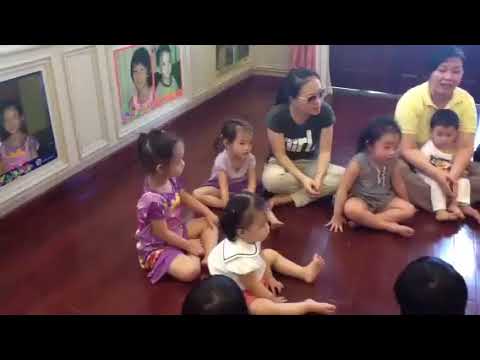This photographic image captures a cozy living room scene with two adult women and five or six barefoot children, all sitting cross-legged on a shiny, red hardwood floor. The group is arranged in a semicircle, facing an unseen focal point in the center. One of the women, who has short black hair and wears a yellow t-shirt, cradles a little boy dressed in white. To her left, another woman wears a black t-shirt with unreadable lettering and light-colored pants. The children, whose dark hair is styled with ponytails, are also barefoot and dressed in various clothing, including a girl in a gray top with drawstrings, a girl wearing a purple dress, and another child in a white and purple shirt. An Asian child is among them, adding to the group’s diversity.

In the background, a white wall decorated with framed photos of a mother and child adds a personal touch to the setting. Two shadows from unseen observers in the foreground suggest the presence of more people outside the frame. A thick black border on the top and bottom accentuates the image. To the upper right of the frame, a closed doorway is visible, hinting at other parts of the home. This intimate snapshot seems to capture a moment of shared attention and community.